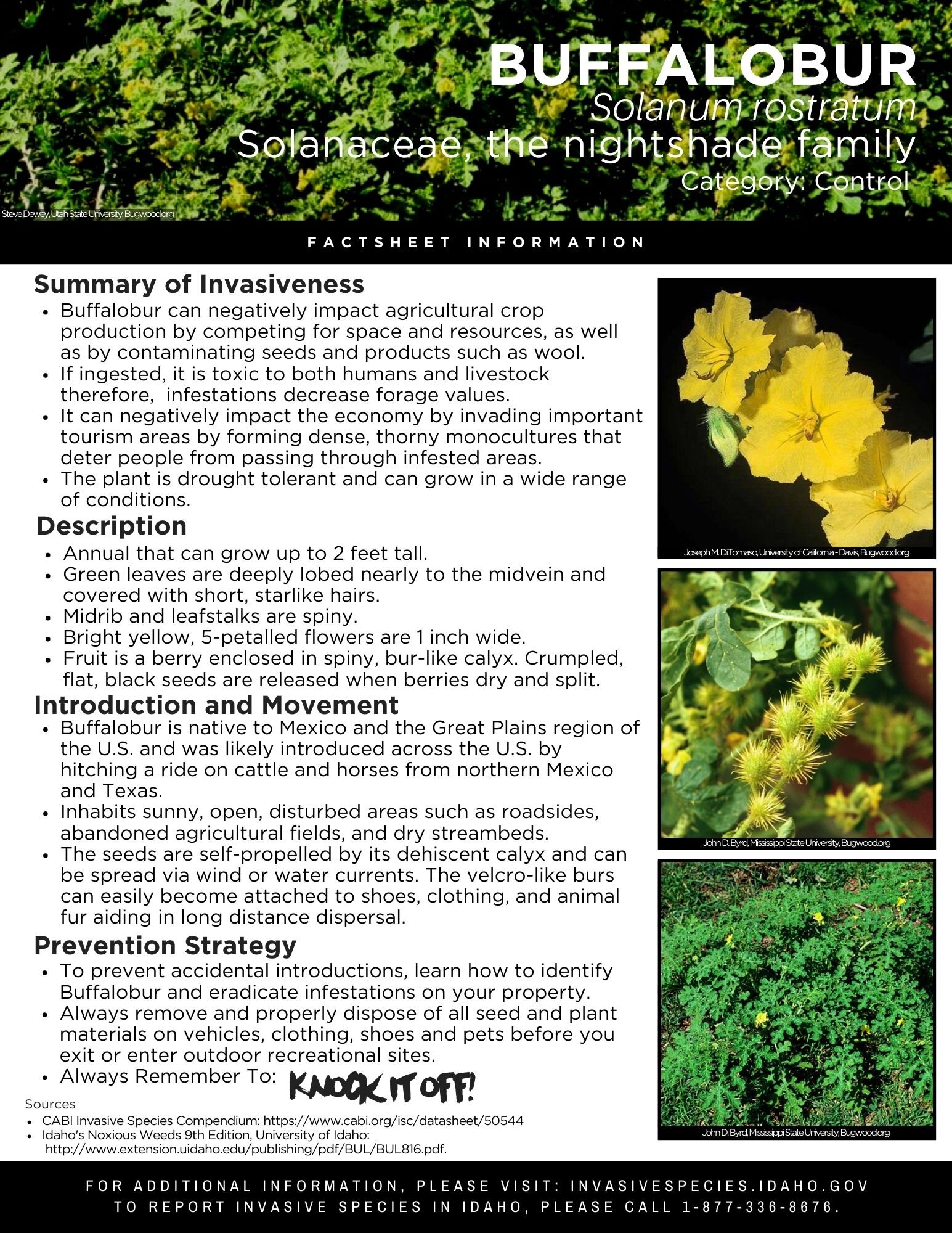The image is a detailed informational brochure about Buffalo Burr (Solanum rostratum), a member of the nightshade family. At the top, the brochure highlights its classification within the Solanaceae family. The document is titled "Category Control" and features a "Summary of Invasiveness" fact sheet. It explains that Buffalo Burr negatively impacts agricultural crop production by competing for space and resources, and contaminating seeds and products like wool. It is toxic to both humans and livestock, decreasing forage value. Economically, it disrupts tourism by forming dense, thorny monocultures that deter passage. The plant is drought-tolerant and grows up to two feet tall in various conditions. The brochure provides images of the plant, showing its distinctive features, including yellow flowers and spiky foliage. Additional sections cover its introduction and movement, detailed descriptions, and preventive strategies with the tagline "Knock It Off." It advises visiting a specific Idaho government website or calling a hotline to report infestations and offers tips for eradication.